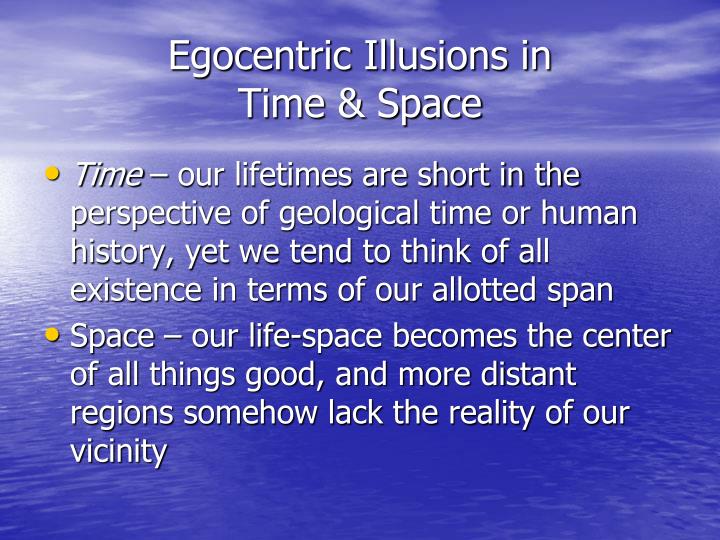The image features a slide from a scientific slideshow presentation, depicting a tranquil blue horizon where the sky meets the ocean. Sparse white clouds adorn the sky, while the sun reflects off the left side of the water, adding a serene touch. Centered at the top of the image in white text, the title reads "Egocentric Illusions in Time and Space," divided into two rows. Below the title, two yellow bullet points are presented. The first bullet point reads, "Time—Our lifetimes are short in the perspective of geological time or human history, yet we tend to think of all existence in terms of our allotted span." The second bullet point states, "Space—Our life space becomes the center of all things good, and more distant regions somehow lack the reality of our vicinity." The detailed juxtaposition of text and a subtly crafted computer graphic background illustrates the thematic exploration of temporal and spatial egocentric illusions.